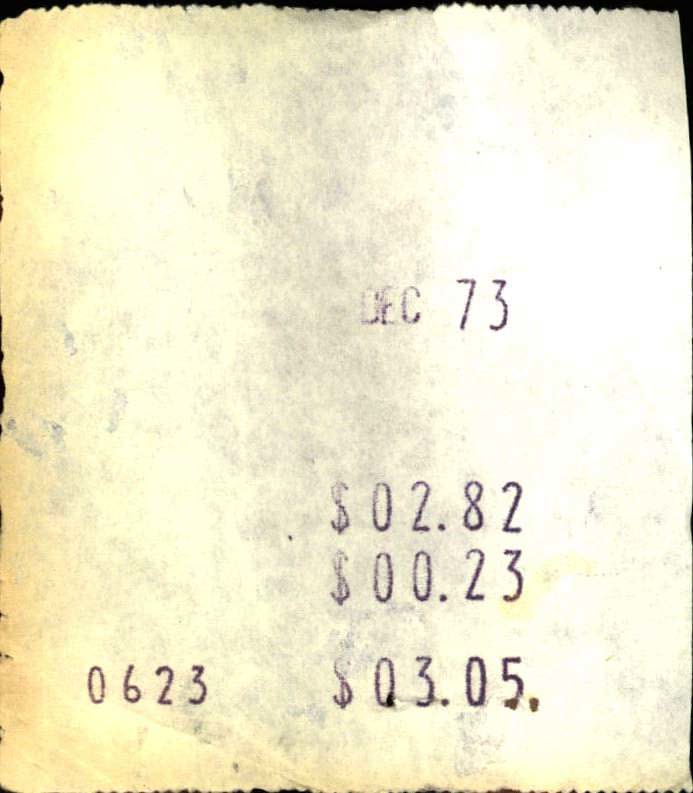This close-up photograph captures a very worn and ragged old receipt, likely from December 1973, as indicated by the faded print "DEC 73" slightly above the center of the page. The receipt appears to have been left out in the sun, leading to its severely faded and yellowed condition, with edges that are serrated and somewhat irregular. The paper, originally white, has darkened to a solarized tan-yello sh hue with black and grayish smudges, indicating significant age and wear.

Positioned on a black surface, the receipt shows various monetary amounts printed in a deteriorated fashion. Specifically, along the right side from the bottom upward, there are three separate lines with dollar amounts: $3.05, $0.23, and $2.82. Additionally, the left side of the receipt near the bottom features the number "0623," which could pertain to a store or transaction number. Overall, the image highlights the effects of time on paper, displaying a snapshot of a bygone era through this tattered financial relic.